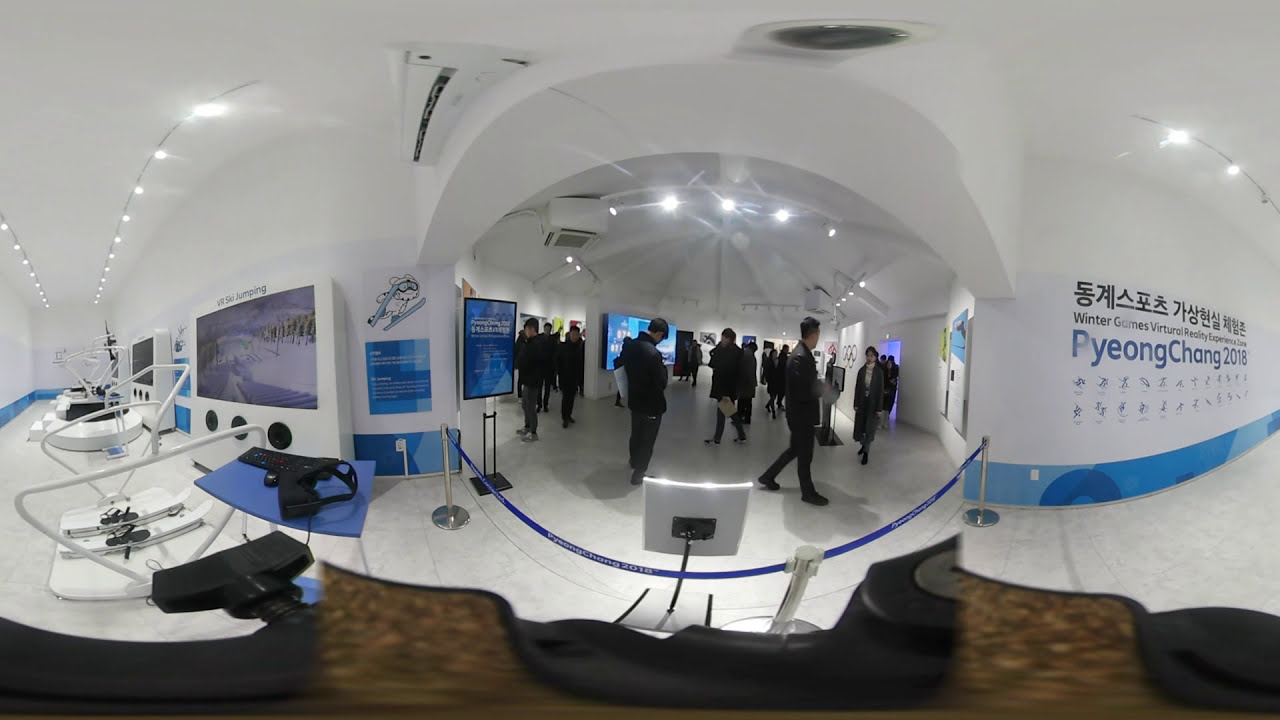The image depicts a large, white-walled museum hall showcasing a "PyeongChang 2018 Winter Games Virtual Reality Experience Zone." The scene is captured with a fisheye lens, adding a subtle dome-shaped distortion to the visual. In the spacious central room, around 20 visitors, predominantly dressed in black coats, are seen walking around and interacting with various exhibits and displays. These include devices like keyboards set on tables and multiple monitors on the walls. There are also visible signs indicating "VR Ski Jumping" among other virtual reality experiences. The environment is brightly lit with fluorescent lights, and the overall atmosphere suggests a high-tech, immersive experience possibly linked to a video game convention or a special event dedicated to the Winter Olympics of 2018 held in PyeongChang. Notably, the presence of Chinese lettering and the predominantly Asian crowd suggest that the museum may be located in China. Two hallways extend from the central area toward the left and right, but access to these passages is restricted by blue ribbons.